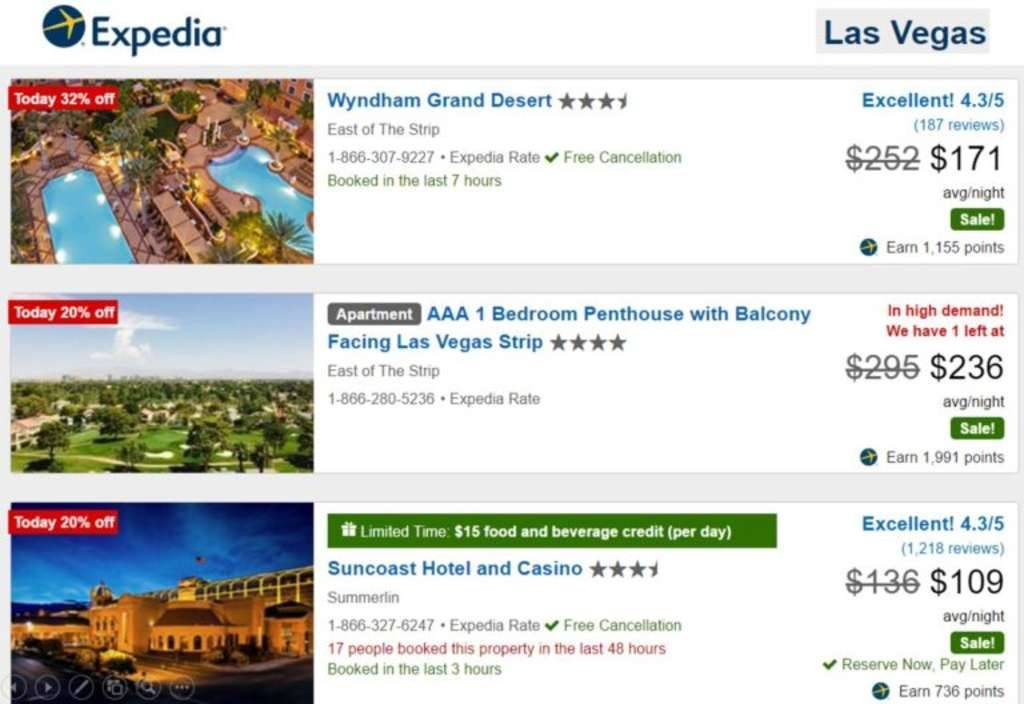This image appears to be a screenshot from the Expedia website. In the top left corner, there's a blue circle with a yellow airplane icon, next to the word "Expedia" in bold letters. On the top right corner, a small gray rectangle contains the text "Las Vegas" in dark blue.

Below this header, the webpage showcases three different vacation options with accompanying images. 

1. **Wyndham Grand Desert:**
   - **Image:** Features two adjacent swimming pools.
   - **Promotion:** "Today 32% off" banner at the top.
   - **Details:**
     - Location: East of the Strip.
     - Rating: "Excellent" 4.3 out of 5 from 187 reviews.
     - Price: $171 average per night.
     - CTA: Green "Sale" button.

2. **AAA One-Bedroom Penthouse:**
   - **Image:** Depicts houses on a golf course.
   - **Details:**
     - Accommodation: One-bedroom penthouse with a balcony facing the Las Vegas Strip.
     - Urgency: "In high demand, we have one left."
     - Price: $236 average per night.
     - CTA: Green "Sale" button.

3. **Suncoast Hotel and Casino:**
   - **Image:** Showcases the exterior of the hotel.
   - **Promotion:** Green banner stating "Limited time $15 food and beverage credit per day."
   - **Details:**
     - Rating: "Excellent" 4.3 out of 5 from 1,218 reviews.
     - Price: $109 average per night.
     - CTA: Green "Sale" button with a check mark and "Reserve now, pay later."

Each option also provides phone numbers for bookings and information about points earned from Expedia at the bottom.